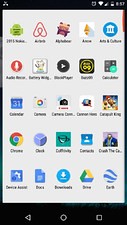A screenshot of a smartphone's home screen displays a grid of apps against a background bordered by thin black margins on all sides—the top and sides featuring the thinnest borders and a slightly thicker one at the bottom. At the top, the status bar shows essential information, including the time (8:57), Wi-Fi connection, and remaining battery life. 

Beneath this, the screen is filled with a 6x5 grid of app icons. The first row from left to right includes a green robot icon (presumably for Android), a purple "A," a bear-like icon, a white square with a yellow center, and a blue circle with a white building. The next five rows continue this pattern, though specific app details aren't entirely recognizable. Among these icons, familiar apps such as music players, Chrome, and email clients are present.

At the bottom of the screen, navigation icons are displayed on a black background: a white outline of a left-pointing arrow on the left, a white circle in the center, and a white square outline on the right.